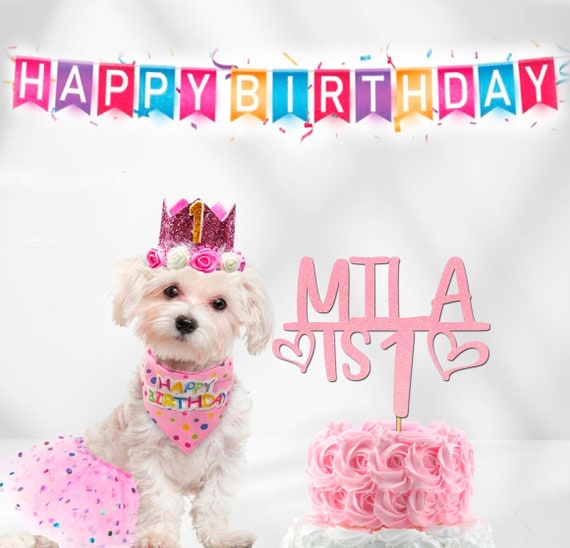This square image celebrates a dog's birthday with a white background. At the top, a colorful banner with alternating rainbow-colored letters spells out "Happy Birthday," adorned with confetti and streamers. Below, to the left, is an adorable small terrier-like dog with medium-length white fur, cute black eyes, and a black nose. The dog wears a glittery pink princess crown decorated with white and pink roses. Around its neck is a pink bandana with a colorful polka dot pattern, proclaiming "Happy Birthday" in alternating rainbow colors. The dog is also dressed in a pink tutu with multi-colored polka dots. Seated on its haunches, the dog's two front paws are visible on the ground. To the right of the dog is a beautiful two-layer birthday cake; the bottom layer is white, and the smaller top layer is pink, decorated with large swirled icing resembling carnation flowers. A sign stuck into the cake reads "Mila is one," decorated with little pink hearts and glitter.